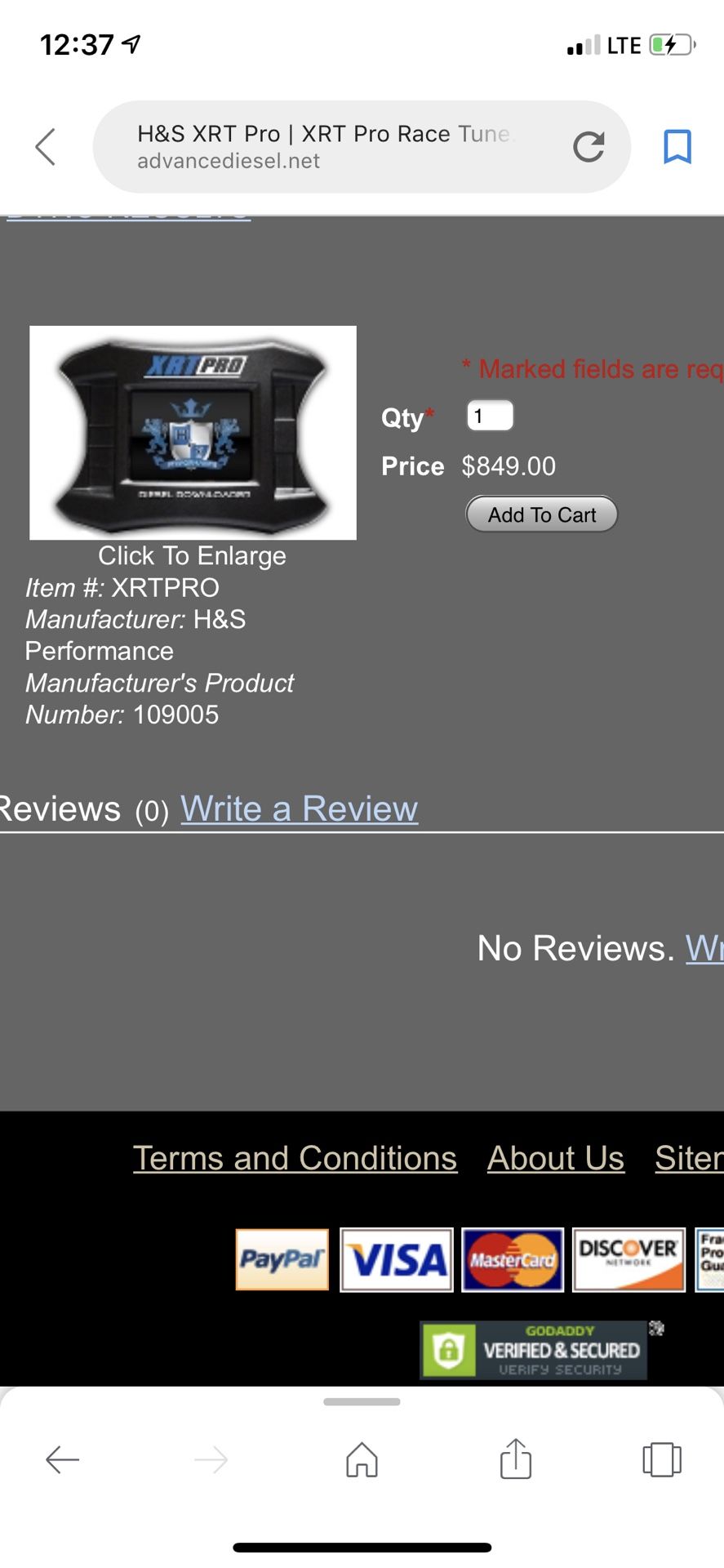Screenshot Description: 

The screenshot appears to be taken from a smartphone displaying a product page from AdvancedDiesel.net. The interface features a predominantly gray upper section and a black lower section.

At the very top, it is 12:37 PM next to a black arrow on the upper left corner. On the right, there are Wi-Fi indicators and battery status symbols. Below this, there are navigation elements, including arrows and labels such as "H", "S", "X", "R", "T", "Pro", "Line", and "X", "R", "T", "Pro", "Race", "Tune". 

A search bar with an arrow in it, presumably to initiate a search, is outlined in blue, suggesting an option to save or mark the website. Below this is a gray area containing product details: the product itself (though unspecified), its item number, the manufacturer, performance details, and the manufacturer's product number are listed. 

To the right of the product description, the quantity is indicated as "1" with a price of $848.49. An "Add to Cart" button is prominently displayed, followed by a "Reviews" section indicating no current reviews with an option to "Write a review" highlighted in light blue.

The background then transitions to black, listing sections like "Returns and Conditions" and "About Us", although parts of these sections are cut off. There are icons for various payment options including PayPal, Visa, MasterCard, Discover, and others which are partially obscured.

At the bottom, there are indications of security features such as a "Verified and Secure" label and the GoDaddy logo accompanied by a lock symbol.